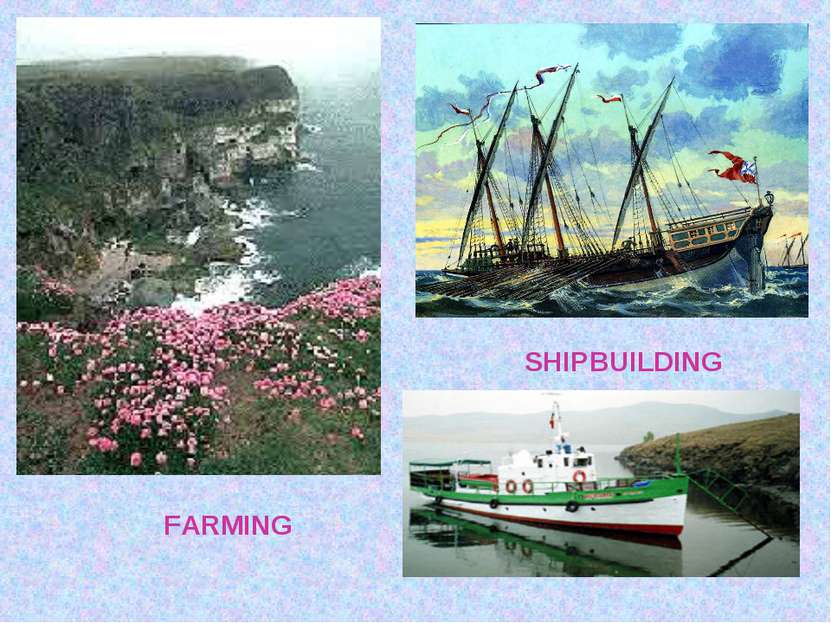This composite image, resembling a PowerPoint slide, is divided into three sections. The left-hand side features a tall, vertically oriented photograph capturing a dramatic coastal scene. Here, one can see a steep rocky cliff plunging into crashing ocean waves below. At the top of the cliff, pink flowers dot the landscape amid dark green foliage. The text "farming" is displayed in purple at the bottom of this image.

On the right-hand side, two images are stacked vertically. The top image is a detailed illustration of an old-fashioned sailing ship with numerous oars and red flags, battling through rough, choppy waters. Below it, an actual photograph shows a modern tugboat with a green, white, and red hull pulling into a calm bay. Situated between these two right-side images, the text "shipbuilding" is presented in purple.

The scene, rich in hues including purple, pink, blue, green, gray, white, and black, appears to be part of an educational presentation, emphasizing the themes of farming and shipbuilding through its harmonious yet striking arrangement of visuals.